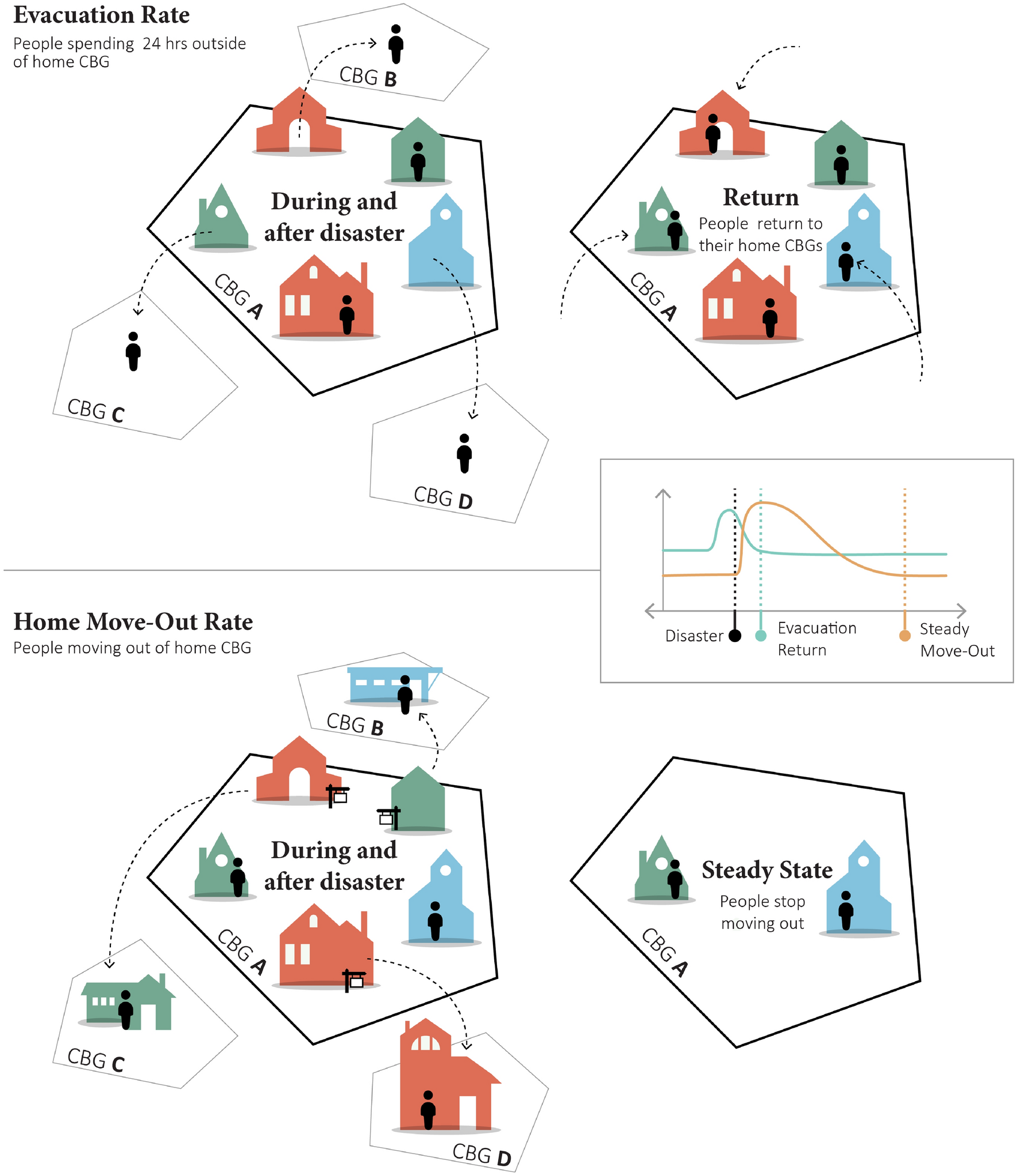The diagram is set against a white background and features four interconnected hexagons and a central rectangle. At the top, the text reads, "Evacuation Rate: People Spending 24 Hours Outside of Home CBG." Within the central rectangle, there are houses labeled "During and After Disaster," with lines extending to smaller polygons outside the main area, each containing a person. 

To the right, another hexagon is labeled "Return: People Return to Their Home CBGs," depicting the reintegration process. Below, a section displays a line chart with a red and blue line, titled "Home Move Out Rate," showing "People Moving Out of Home CBG" and indicating patterns "During and After Disaster." 

The bottom line of the diagram features hexagons labeled "Move Home" and "Move Out Rate," illustrating the transition phases. The last hexagon is tagged "Steady State: People Stop Moving Out," indicating the cessation of evacuation movements. Each hexagon contains houses and figures, depicting various states of occupancy and movement during and after a disaster situation.